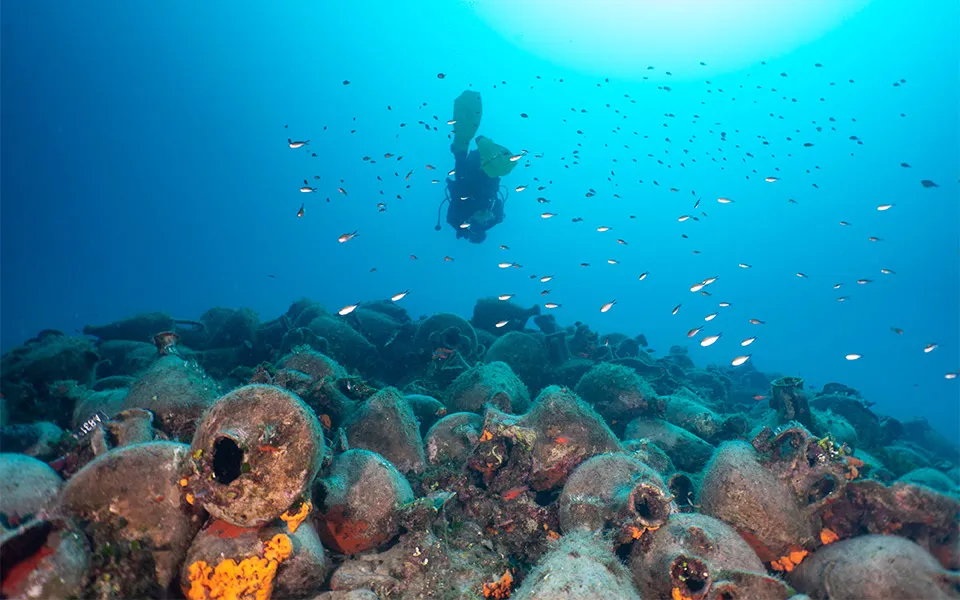A detailed underwater image captures the mesmerizing scene of a scuba diver swimming away from the camera, showcasing only his back adorned with yellow fins and cords extending from his gear. The diver is surrounded by a small school of silver fish, adding a dynamic element to the serene surroundings. The clear, blue waters gradient into turquoise near the surface, where rays of light penetrate the depths. Below, the ocean floor is scattered with amphorae—ancient clay pots and vases, some of which have become coralized with gray hues accented by hints of yellow and orange. This archaeological site, part of the wreck of the ancient Greek ship Peristera, lies 92 feet below the surface off the coast of the island of Alonissos in the Aegean Sea. The image beautifully captures both the mystery of the ancient wreck and the vibrant marine life that has made it a habitat.